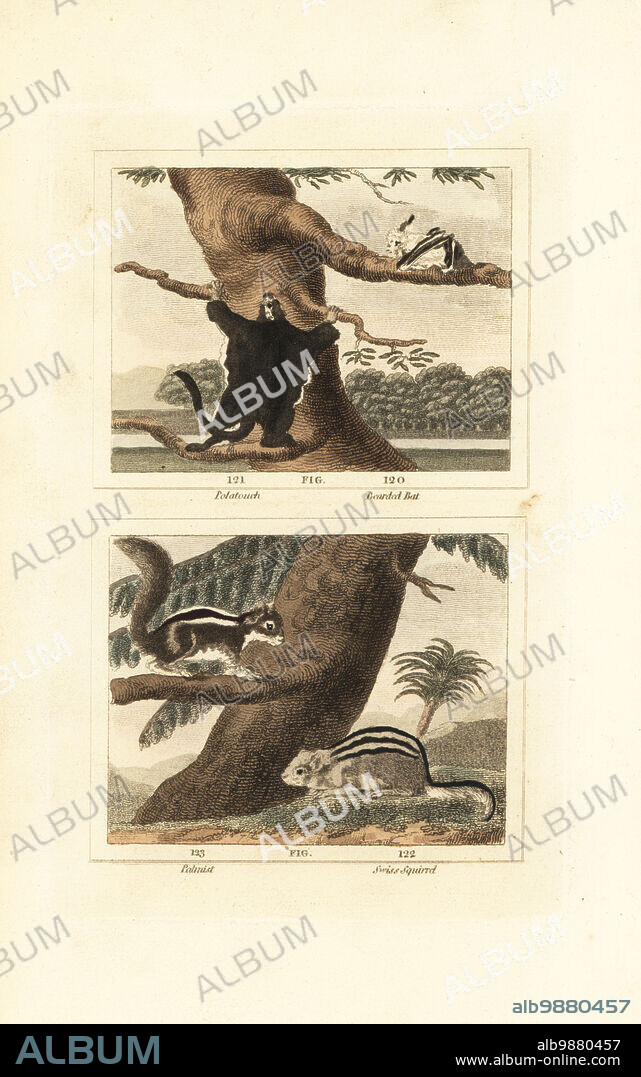The image comprises two diagram-like photographs, prominently watermarked with the word "album." Each photo, arranged vertically on a whitish-pink background, features a tree as the focal point. In the top photograph, a bear stands on its hind legs in front of the tree with its arms extended. The bottom photograph depicts a slanted tree with a palm tree in the background. On the tree, a black and white skunk perches on a branch, looking down at another skunk positioned on a rock at the base. The entire image is stamped with the word "album" and includes a serial number, "ALB 9880457," alongside the website URL "www.album-online.com" in white text at the bottom.